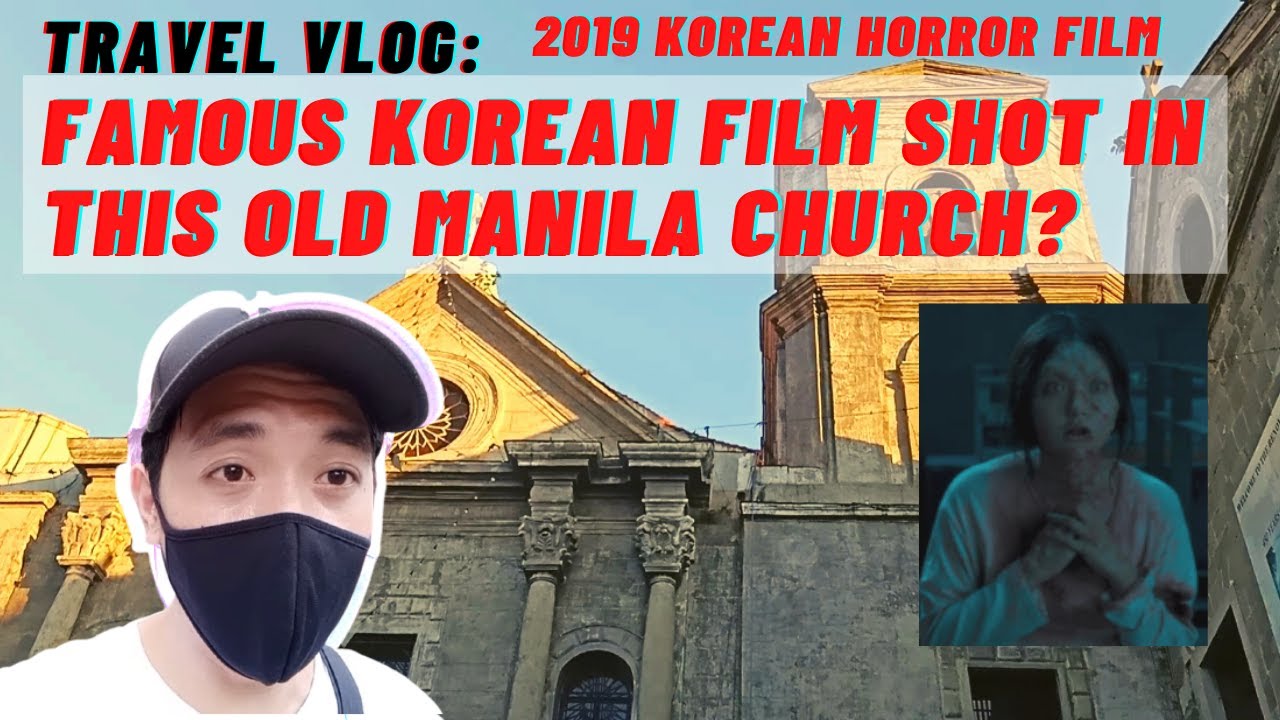In this image, the background features the top of an old church with tan-colored walls, partially illuminated by sunlight, while the lower portion is densely shadowed. The church's architectural details include a central tower with pillars and windows barely visible at the bottom. A clear blue sky with no clouds completes the backdrop.

At the top of the image, black text reads "Travel Vlog," followed by "2019 Korean Horror Film" and "Famous Korean Film Shot in This Old Manila Church?" both in larger red font.

In the foreground, the bottom left corner shows an Asian male with scrunched-up eyebrows, wearing a black face mask, a black baseball cap, and a white shirt. His face appears digitally added with a faint white border along its edges. On the bottom right is a photograph of a woman, covered in blood, her mouth open in a look of horror or surprise. She has dark, shoulder-length hair parted in the center, and blue-toned skin with visible scars, giving her a zombie-like appearance.